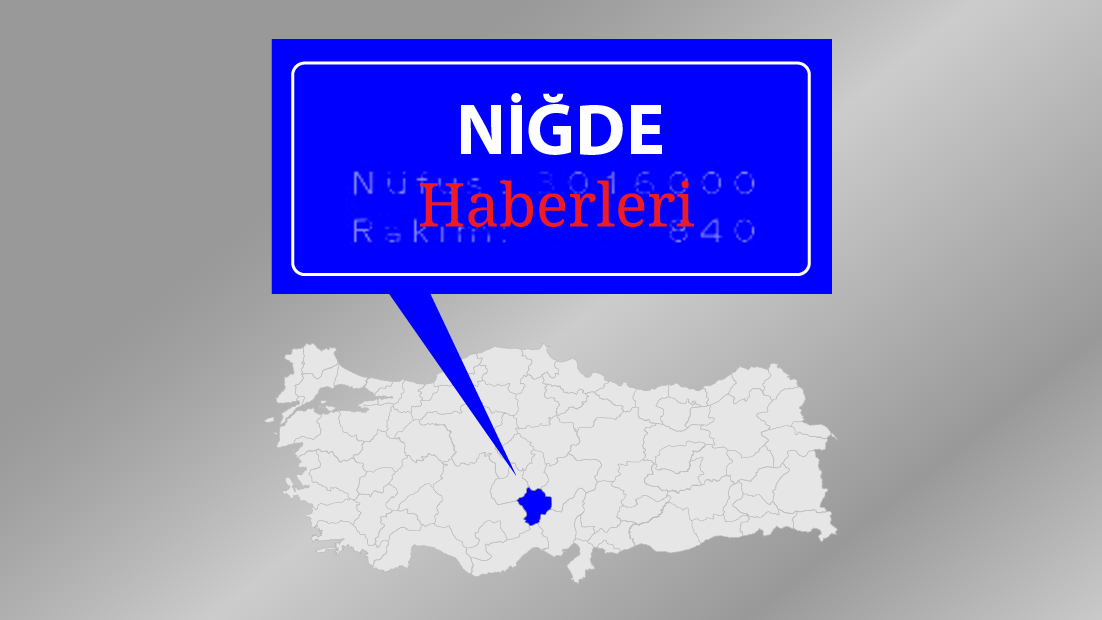The image appears to depict a map of Turkey with a specific emphasis on the province of Niğde. The background is a textured gray, and the country of Turkey is divided into sections by gray lines. The province of Niğde is highlighted, with a blue arrow or pointer directing attention toward it. Over this highlighted section is a blue speech bubble containing the text "NİĞDE" in prominent white letters. Below this, in red letters, it reads "HABERLERİ." Additionally, there are faded white letters in the background that seem to spell out "Nafas Rakhiliya," although these are difficult to read clearly. To the right of the main text, the numbers "3016000" and "840" are also visible in faded white letters. The overall appearance suggests that the image functions as a detailed and annotated map, emphasizing the region of Niğde within Turkey.